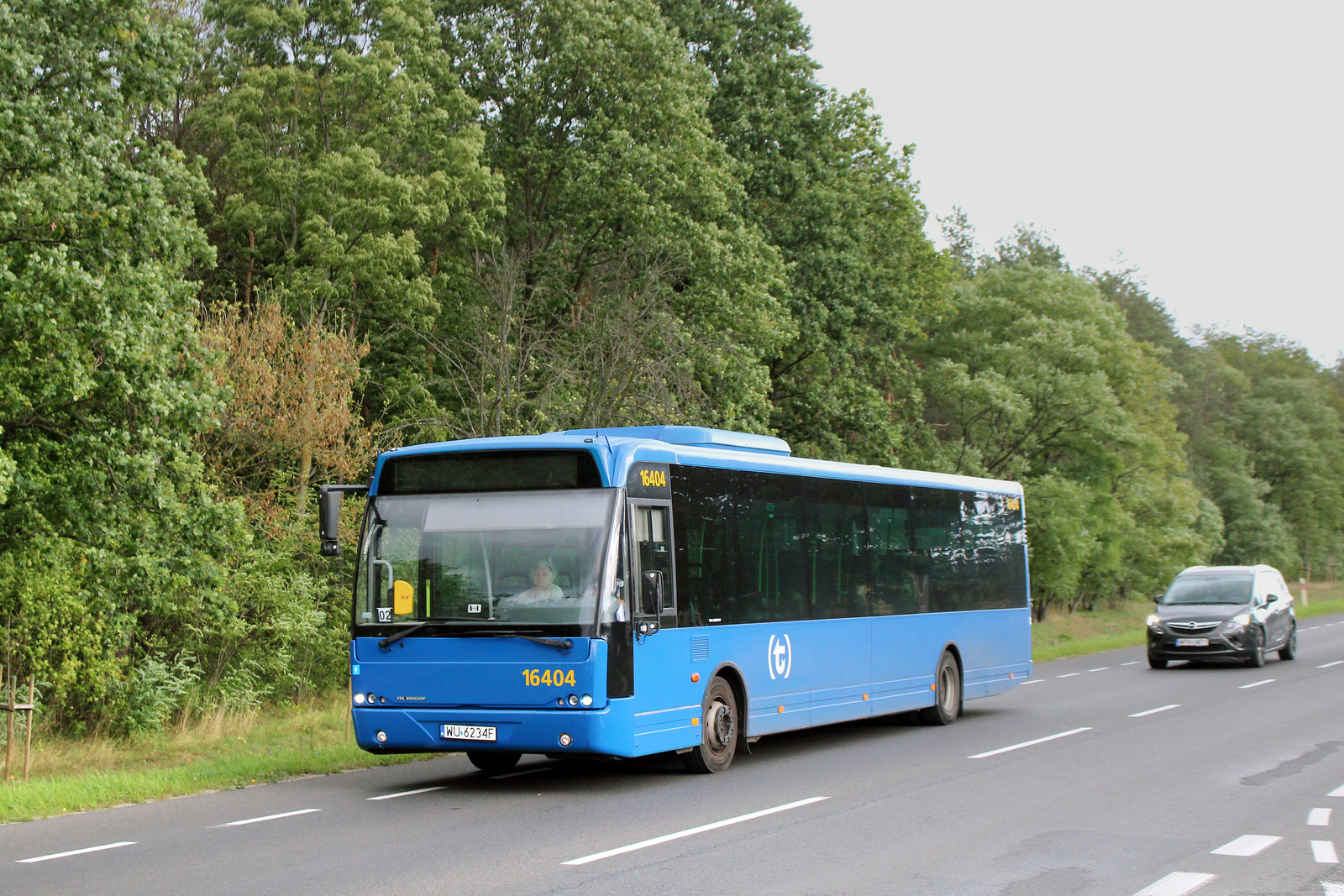In this detailed photograph, we see a vivid blue city bus with large, black-tinted windows, prominently displaying the number 16404 along with a lowercase "T" in parentheses on its side. Through the front window, an elderly woman with gray hair, dressed in a white shirt, is visibly seated. The bus appears to be pulled over slightly in the right lane of a freshly paved road, which runs diagonally from the left towards the bottom of the image. Behind the bus, in the same lane, there is a small, black sedan that seems poised to overtake it. The scene is set against a backdrop of tall, verdant deciduous trees, and the sky overhead is overcast with gray clouds, indicating a cloudy day. The road itself is immaculate and free of cracks, enhancing the contrast between the man-made and natural elements in the image. The license plate on the bus reads WU-6234F, typical of a European style with a white background and a blue area on the left side.